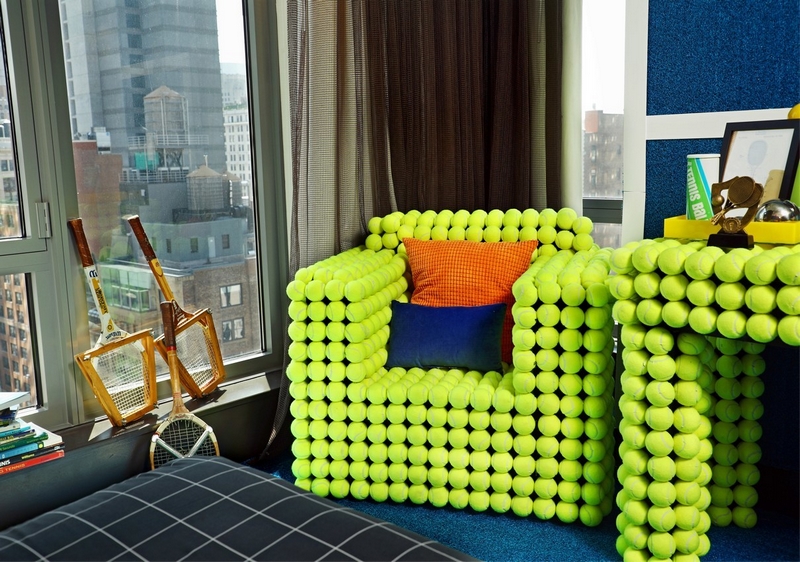The image captures an intriguing scene inside a high-rise condo, showcasing a unique blend of furniture and sports elements. Dominating the foreground is an unusual chair made entirely of stacked tennis balls, with each armrest composed of four tennis balls in width and five in height, while the seat spans approximately ten tennis balls across. It features two pillows, one small and blue, and another orange, balanced against the headrest—though it doesn't look particularly comfy. Adjacent to this chair is a table, also constructed from tennis balls, holding a picture frame and a few knick-knacks.

The setting includes a grid-patterned blue sofa with white marks on its seat part, accompanied by a turquoise blue rug. To the left and rear of the scene, floor-to-ceiling windows reveal a cityscape. A ledge runs along the floor, where three tennis rackets rest against the window, and beside them lies a pile of books. Centrally, a tannish drapery hangs vertically, adding to the room's eclectic decor. The overall atmosphere is a creative and whimsical mix of athletic themes and urban living.